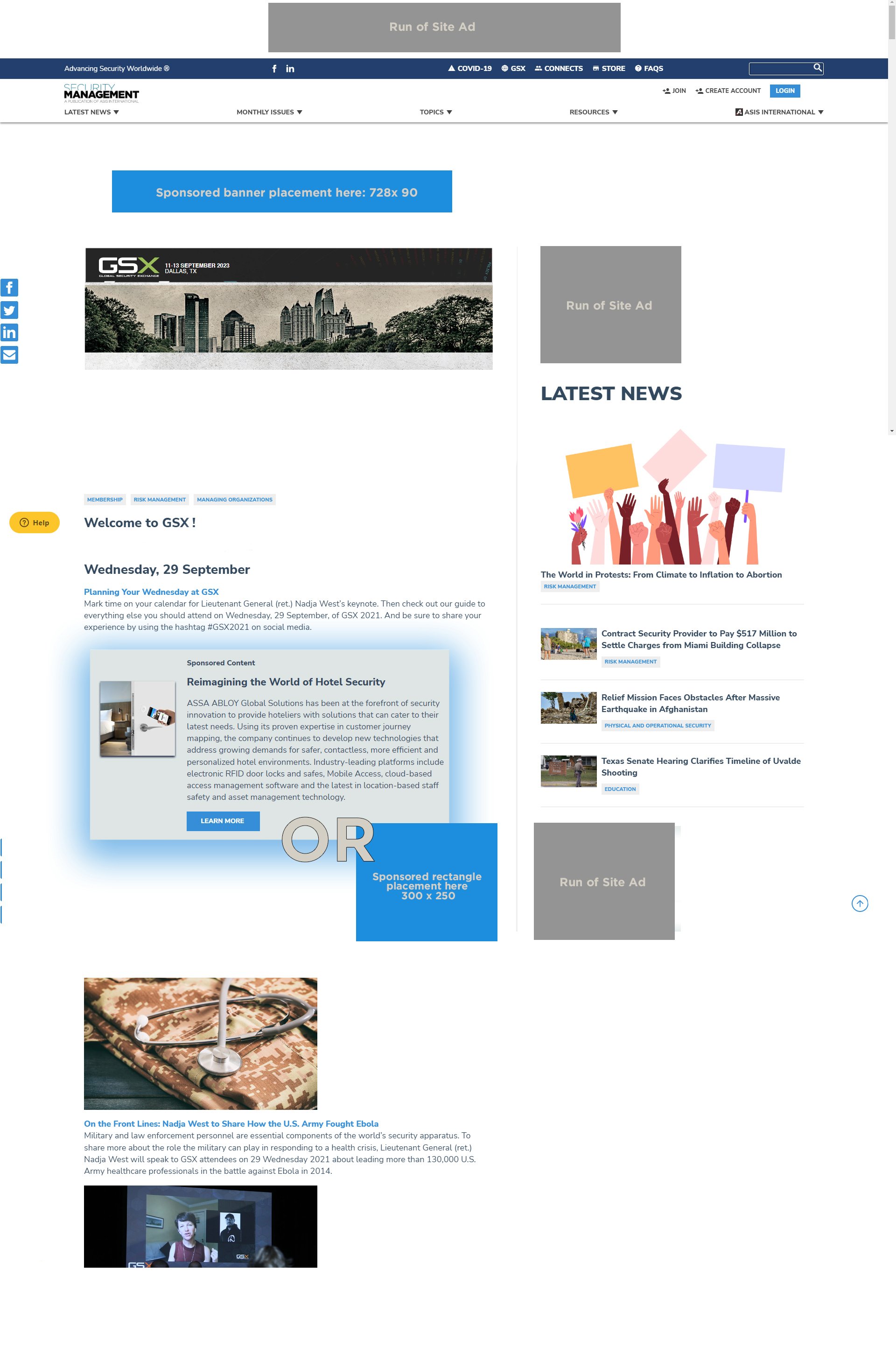The image appears to be a webpage with a focus on GSX Management, specifically titled "Security Management." The text on the page is quite small, but it welcomes visitors to GSX and highlights an event: "Planning Your Wednesday at GSX - Reimagining the World of Hotel Security," dated Wednesday, September 29th. This suggests that GSX offers security management solutions tailored to the hospitality industry.

The layout includes a section for the latest news, and navigation tabs are positioned on the left side, offering links to various social media platforms and an email contact. At the top of the page, there's a black-and-white photograph featuring an old-style hotel, adding a vintage feel to the site. Additionally, a rectangular ad space is labeled for site advertisements. Despite the abundance of information, the small text makes it hard to read the finer details.